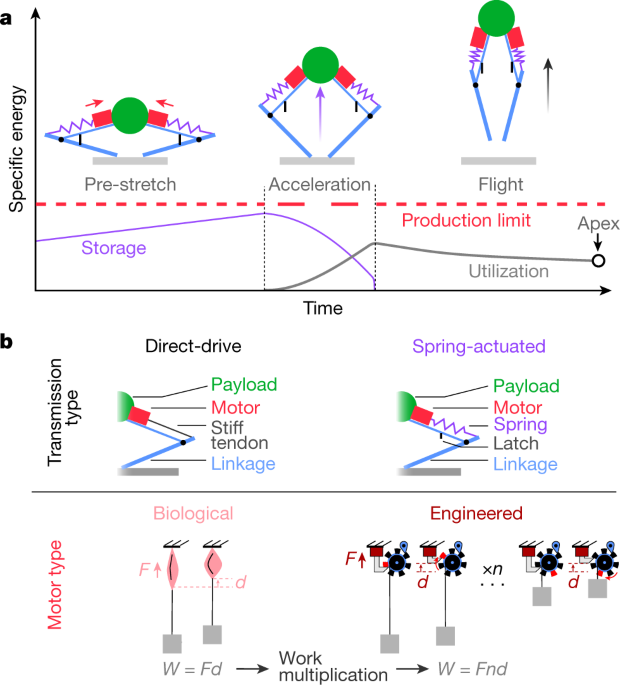The image displays an intricate poster, likely fit for a science classroom or university setting, that is sectioned into two main parts—labeled A and B—to detail different types of energy and mechanisms of action. Part A features a graph with 'specific energy' on the y-axis and 'time' on the x-axis, showing a three-stage process involving 'pre-stretch,' 'acceleration,' and 'flight.' The 'pre-stretch' stage depicts a green circle with red blocks and blue lines, resembling legs or stilts, forming an elongated diamond shape. Red arrows indicate the force direction towards the green circle. The 'acceleration' stage shows this structure lifting, while the 'flight' stage depicts the legs off the ground, with an arrow labeled 'flight' indicating upward motion. Below this graph, the 'storage,' 'timeline,' and 'utilization' are noted, leading to an 'apex' point on the timeline.

Part B explains different transmission and motor types. The 'direct drive' and 'spring actuated' diagrams illustrate the interaction between components like the 'payload' (green circle), 'motor' (red blocks), 'stiff tendon,' and 'linkage' (blue stilt-like legs). The 'spring actuated' version replaces the 'stiff tendon' with 'spring latch' components. Further down, 'motor types' are categorized into 'biological' and 'engineered,' with detailed diagrams showing actuation points and gear work. The poster uses color—predominantly purple and blue—to highlight different energies and their respective processes, making the information visually accessible and highly detailed.